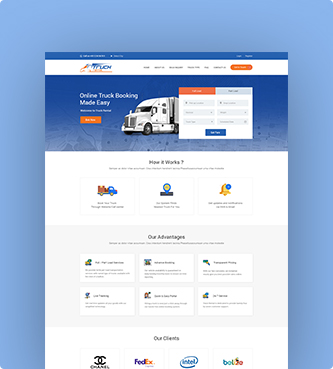This is a screenshot of a website that facilitates easy online truck booking. The design prominently features a large image of an 18-wheeler big rig truck at the top. Below the image, the section appears to explain the process with a heading that likely reads "How It Works," although the text is blurry. The website employs a color scheme of blues, whites, and grays, with eye-catching orange buttons for user interaction. At the bottom of the screen, the logos of FedEx and Intel are visible, indicating potential partnerships or endorsements. The overall layout suggests a professional and user-friendly interface designed to streamline the truck booking process.